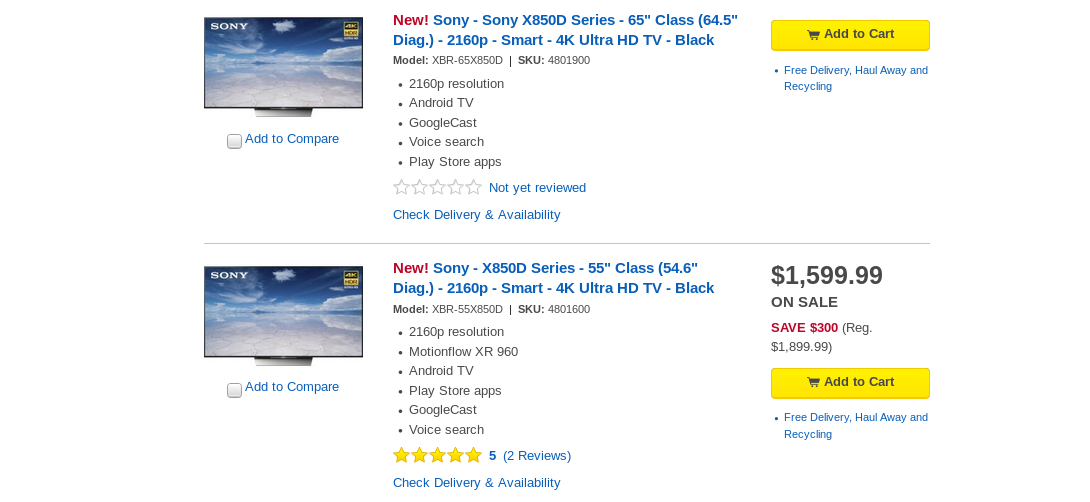This image showcases two Sony monitors displayed vertically, one positioned above the other. Each monitor has an 'Add Card' button prominently featured. The monitors display a scenic image of clouds resembling a serene sky. On both monitors, the brand name "Sony" is prominently displayed in white font at the upper left-hand corner, while a yellowish sticker is noticeable on the upper right-hand corner. Below each monitor, there is a small checkbox labeled "Add to Compare." Despite their similarities in appearance, the top monitor is a 65-inch model and does not have any reviews, whereas the bottom monitor is a 55-inch model and includes customer reviews.